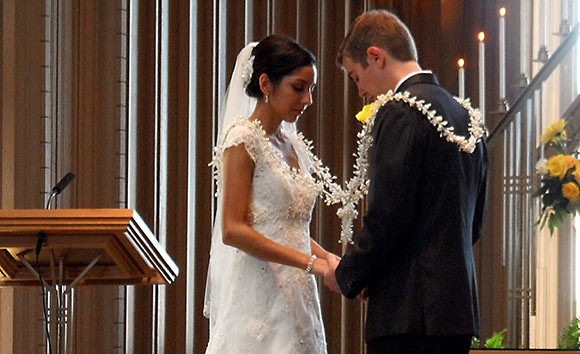In the image of this intimate wedding ceremony, the bride and groom stand at the altar, both deeply focused on their interlaced hands, perhaps exchanging vows. The bride, positioned on the left, is elegantly dressed in a white wedding gown featuring off-the-shoulder, short sleeves with lace detailing. Her hair is styled in a simple low bun adorned with a veil and a delicate flower clip. On her right, the groom is dressed in a classic black suit, complementing the formality of the occasion.

A significant feature of the scene is a large flower necklace or lei draped around both of them, tied in the center above their joined hands, symbolizing their unity. They are facing the camera from the side, making the finer details of their expressions less discernible but highlighting the tenderness of the moment.

To the left of the image stands a podium with a microphone, suggesting the presence of an officiant or speaker. On the opposite side, the right side of the image, is a chapel adorned with candles and flowers in yellow and gold hues, enhancing the sacred and celebratory atmosphere. The decor extends up the side of the wall, adding a warm and festive touch to the ceremony setting.